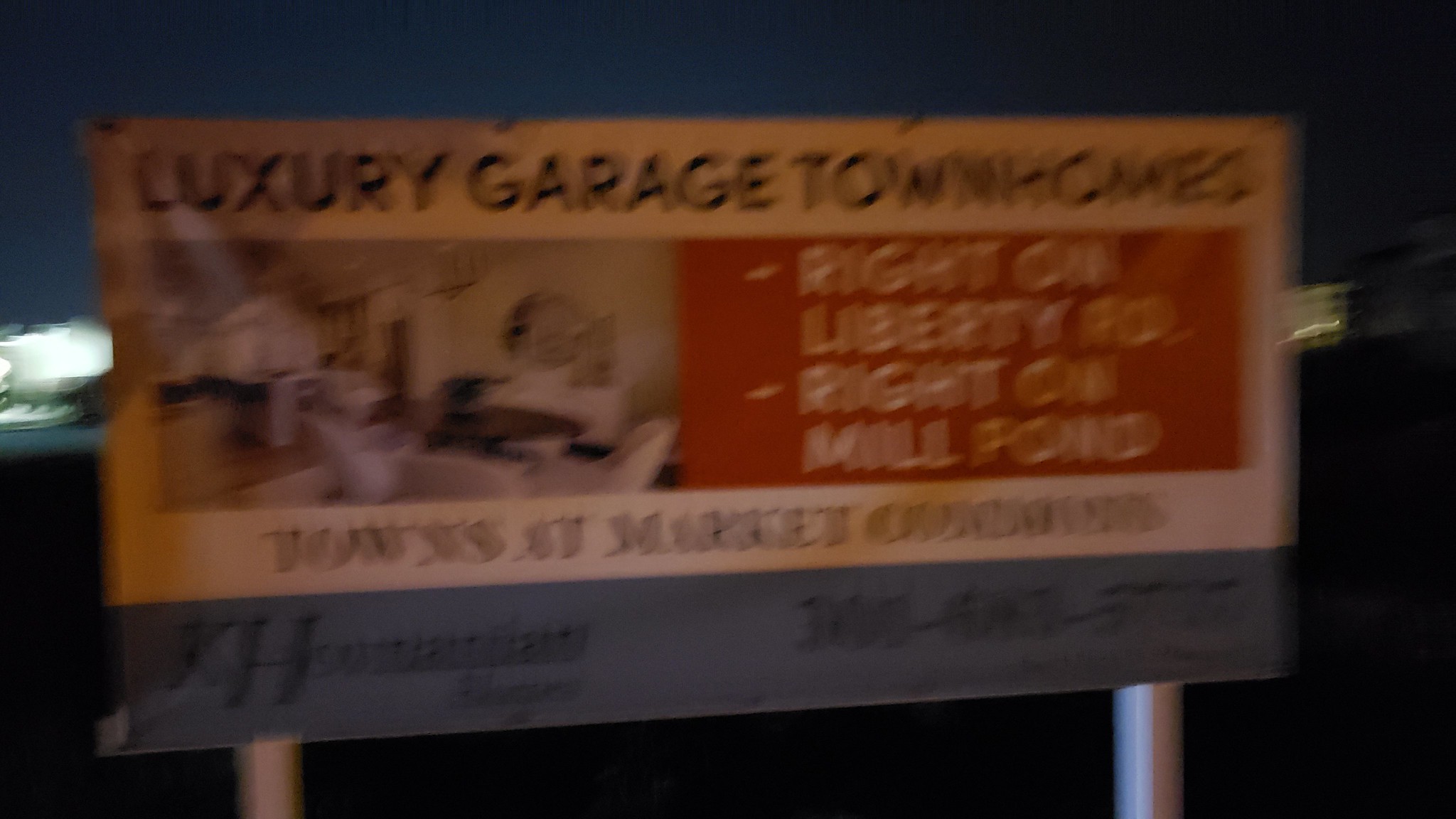A nighttime photograph shows a blurred image of a construction advertisement sign, likely due to unsteady camera movement. The sign, advertising a new home community, is predominantly white on the top and blue on the bottom, where contact information is typically displayed. The upper section features the text "Luxury Garage Townhomes," accompanied by an image of a furnished interior. To the right of the image, the sign reads "Right on Liberty Road, Right on Mill Pond." Below this, the text "Towns at Market Commons" is faintly visible, though slightly obscured by the blur. At the bottom of the sign, it seems to read "Hawaiian Homes," with a phone number to the right that is indistinguishable due to the image's blurriness.